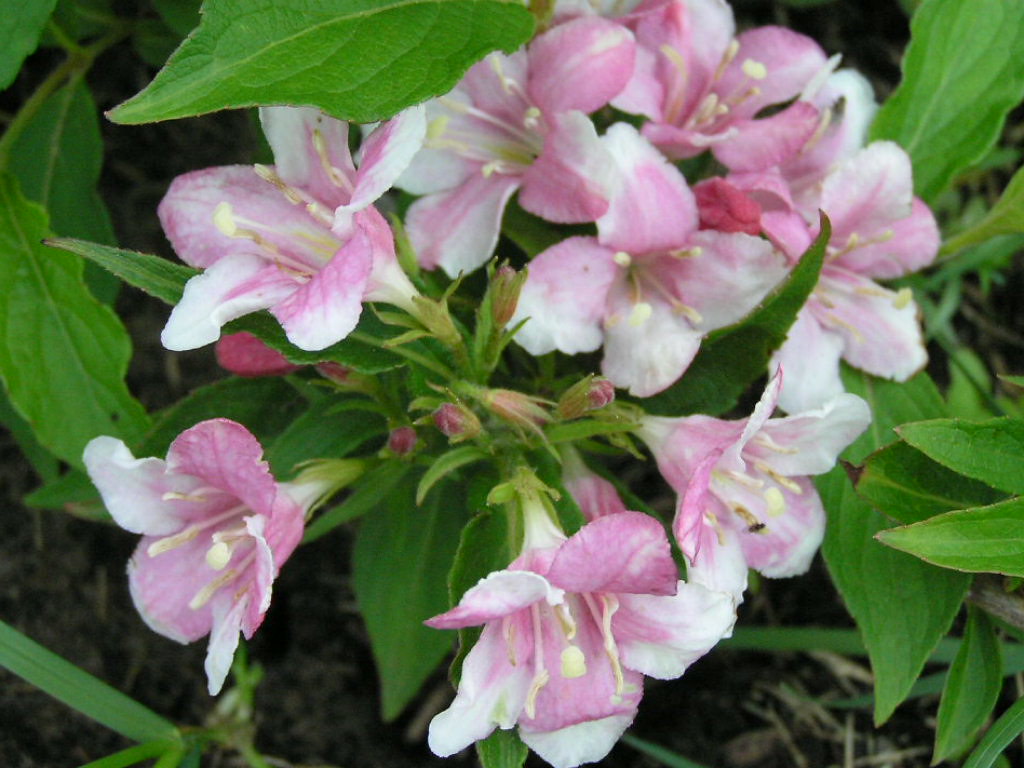The close-up photograph captures a vibrant scene of a wild floral arrangement at the end of a bush’s stem. Dominated by lush green foliage and leaves, the image prominently features an array of pink and white flowers situated primarily in the top middle and cascading down the right side to the bottom middle, with a solitary flower in the bottom left corner. The flowers showcase delicate petals with central pistils or stamens, and each bloom is surrounded by additional buds that are mostly green but hinting at a darker pink hue as they begin to open. Amidst the dense greenery, patches of dirt and sparse grass are visible on the ground, providing a natural background to the blooming cluster of around ten flowers, arranged in a circular pattern with about six or seven partially opened buds in the center. The scene is lively, capturing the essence of nature’s beauty in a detailed and vivid portrayal.